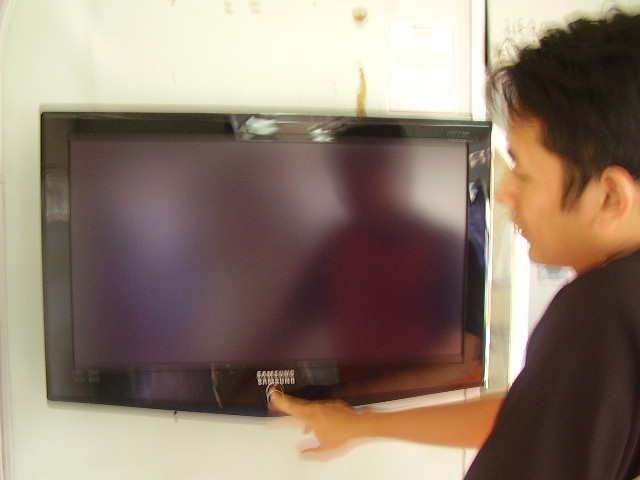In this blurry, indoor photographic image, an Asian man, likely in his thirties or forties, is seen wearing a black short-sleeved shirt. He is standing close to a wall-mounted Samsung television, which is turned off, causing the screen to reflect his silhouette. The man, with short black hair and prominent sideburns reaching down to the base of his ears, has a pointy nose and brownish-yellow skin. He is facing left and is captured in the act of reaching out with his right hand, aiming to press the power button located at the bottom center of the television. The beige wall behind him has some noticeable stains. The photograph is quite blurry, suggesting motion at the time it was taken, resulting in a double image of the Samsung logo and a generally unclear depiction of the scene. The bright room is illuminated by sunlight, adding further glares to the TV screen, enhancing the overall silhouette effect.